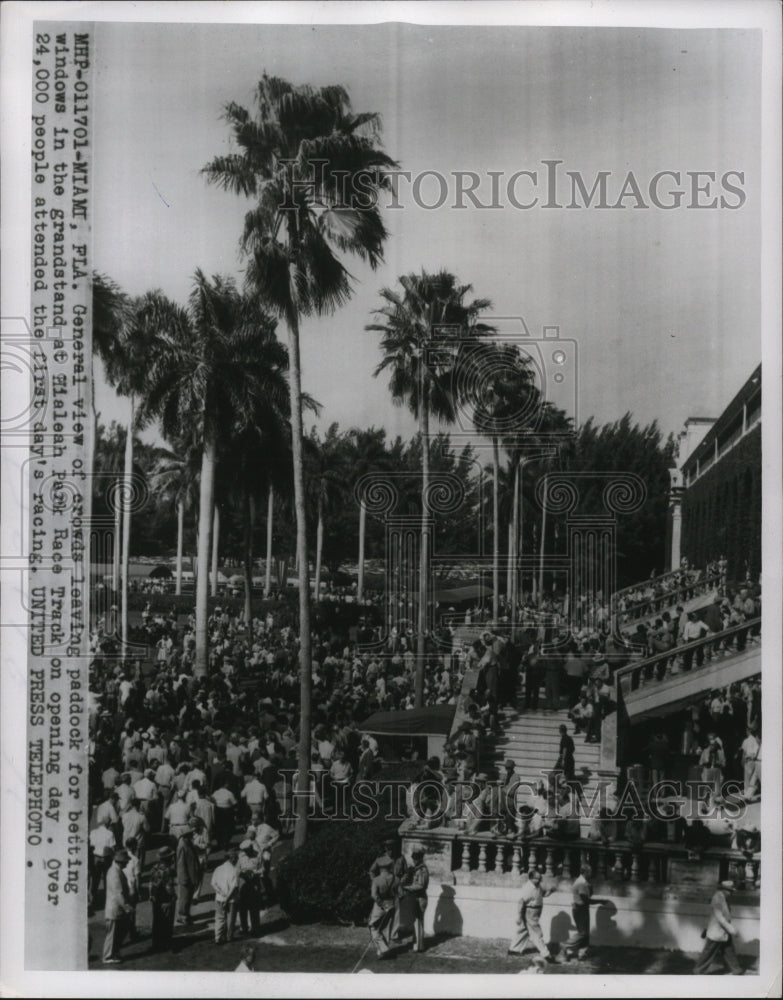The black and white photograph captures a bustling scene at Hialeah Park Racetrack in Miami, Florida on opening day, with over 24,000 attendees. Highlighting natural light, the vertically rectangular image, bordered in light gray, is populated with dozens of people milling about in an open area. Prominent tall palm trees indicate a tropical setting. In the background, there is an ornate staircase on the right with people moving up and down. Various watermarks, including the Historic Images logo—a design featuring an H formed by two pillars and an old-school camera—are spread over the image. Additionally, sideways text along the left edge reads, "MHP-011701-Miami PLA. General view of crowds leaving paddocks for betting windows in the grandstand of Hialeah Park Racetrack on opening day. Over 24,000 people attended the first day's racing. United Press Telegraph." The photograph portrays a lively atmosphere amidst the grandeur of the racetrack on its much-anticipated opening day.